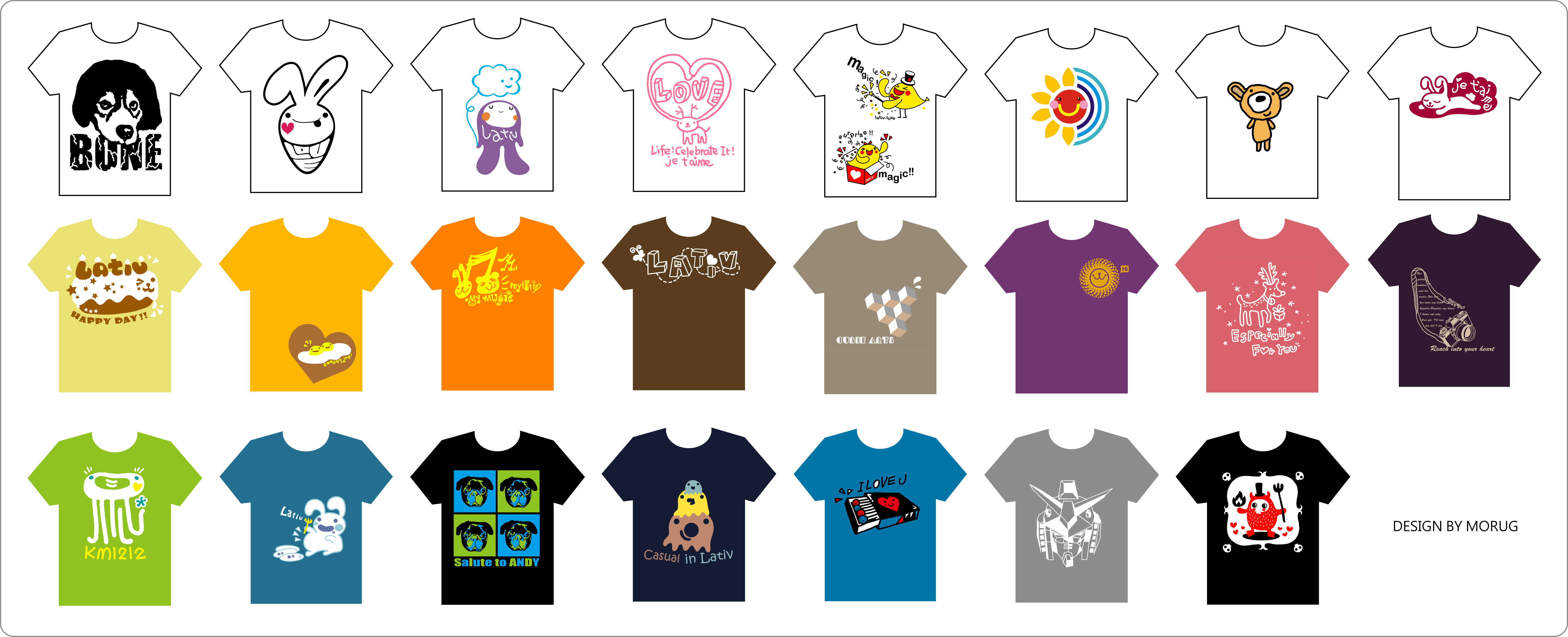The image showcases a digitally created assortment of crewneck, short-sleeved t-shirts displayed against a clean white background, each outlined by a thin black border. The layout features three rows of t-shirts, each adorned with distinctive, cartoon-style designs. The top row consists entirely of white t-shirts featuring black illustrations, including a dog, a bunny shaped like a carrot, the sun, a teddy bear, clouds, a heart, and other whimsical graphics, with one t-shirt displaying the word "bone."

The second row introduces t-shirts in various vibrant colors: yellow, light orange, orange, brown, light brown, purple, light red, and black. Each shirt in this row showcases a unique cartoon image. 

The bottom row continues with an array of colored shirts, including bright green, teal green, blue, dark blue, light blue, gray, and black. These also feature diverse cartoon images, with one notable design being a little demon with a hat on a black t-shirt in the bottom right.

In the corner of the image, it reads "Designed by Mobug," indicating the creator of these playful and varied t-shirt designs. This image appears to be a sample sheet or catalog for a clipart website, offering a glimpse of various designs available for customization.